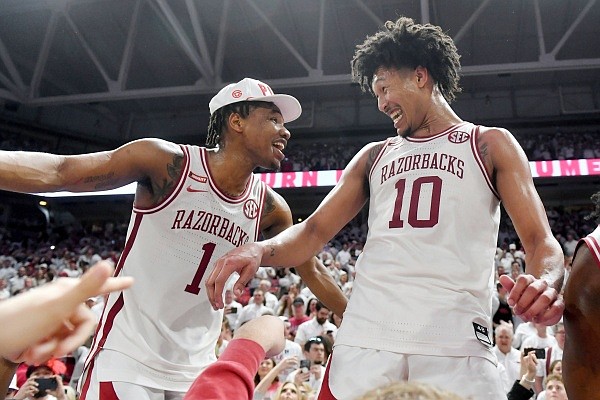In the image, two exuberant basketball players from the Razorbacks team stand inside a covered stadium. The stadium is packed with enthusiastic fans on both the lower and upper levels, visible in the background. The structure's white metal support beams are seen at the top of the frame. 

The player on the left, wearing a white cap and the number one jersey, extends his arms outward and leans towards his teammate on the right. He is smiling broadly, showcasing his teeth, and appears to be celebrating. The player on the right, who has poofy black hair and is number ten, is smiling back at his teammate and appears to be looking down towards him. This player, positioned on our right side of the image, strikes a less exaggerated celebratory pose with his arms slightly out.

Both players are surrounded by a crowd, with numerous hands reaching up towards them from the foreground, hinting at the fans' excitement and admiration. The scene suggests a moment of victory, filled with joy and energy, as the players revel in their triumph amidst a sea of supporters.